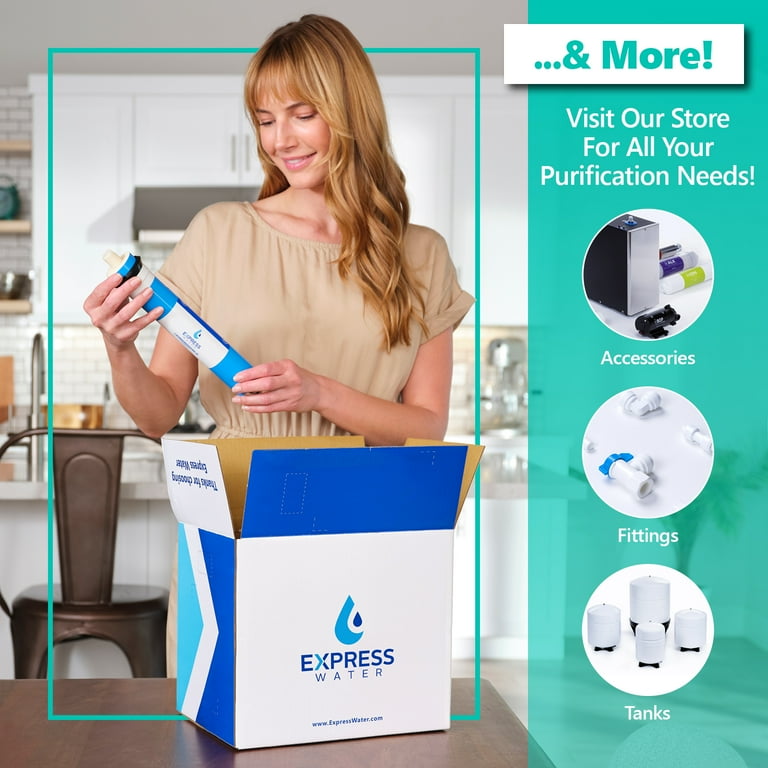This advertisement image features a Caucasian woman with long auburn hair, dressed in a tan dress, standing in her pristine, white-themed kitchen. She is smiling and looking down at a cylindrical water filter she has just pulled out from a blue and white box labeled "Express Water," prominently featuring a water drop logo. The box, which sits on a wooden table, has a multi-colored design with various shades of blue. Behind her, the kitchen boasts white cabinets, white subway tile walls, and a silver stand mixer on the white countertops. A barstool is visible at the countertop, and three wooden shelves to the left display various kitchen items. In the background, against a greenish-blue overlay, the words "Ann Moore" appear, along with a call to action in white lettering: "Visit our store for all your purification needs." Additionally, three white circles beneath the text highlight different product categories: accessories, fittings, and tanks, each accompanied by respective images of these components.